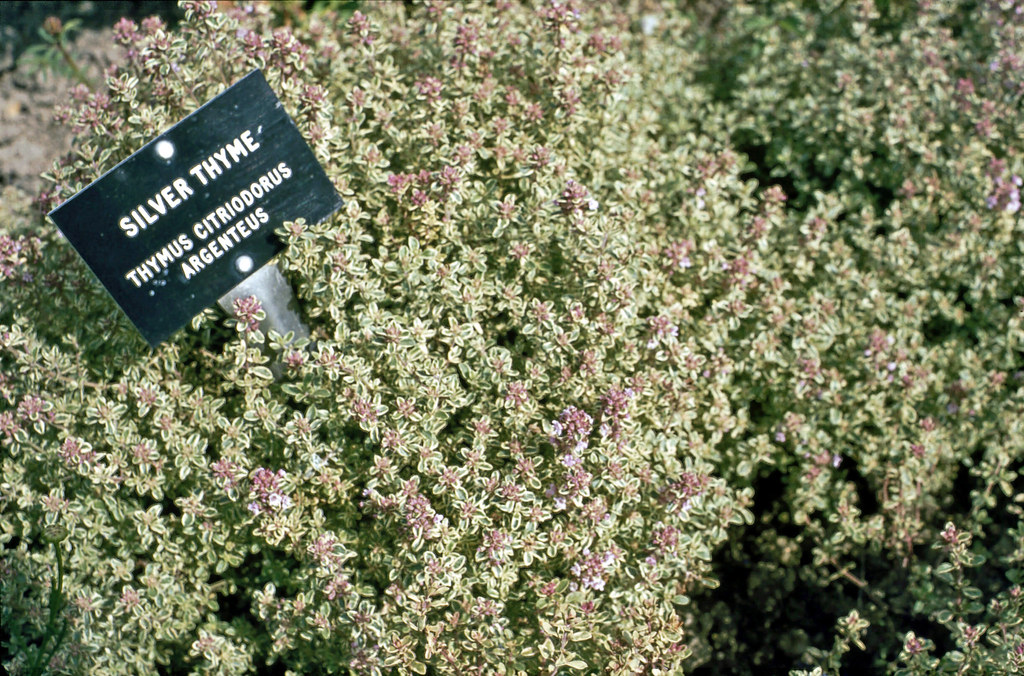This close-up photograph captures a dense and bushy plant, filling the entire frame. The plant, identified as "Silver Thyme" with the scientific name "Thymus Citriodorus Argenteus," is detailed by a black sign with white lettering, positioned diagonally in the upper left corner, secured by two metal screws. The small, delicate flowers are clustered together, displaying a mix of white, green, and pink hues. The foliage consists of dark green, slightly rounded leaves, bordered with a lighter green or yellowish tint, arranged in a layered, alternating pattern, resembling a plus sign structure. Some leaves are topped with tiny purplish flowers. The intricate details of the plant, from the minute leaves to the tiny flowers, emphasize its delicate and ornamental nature.